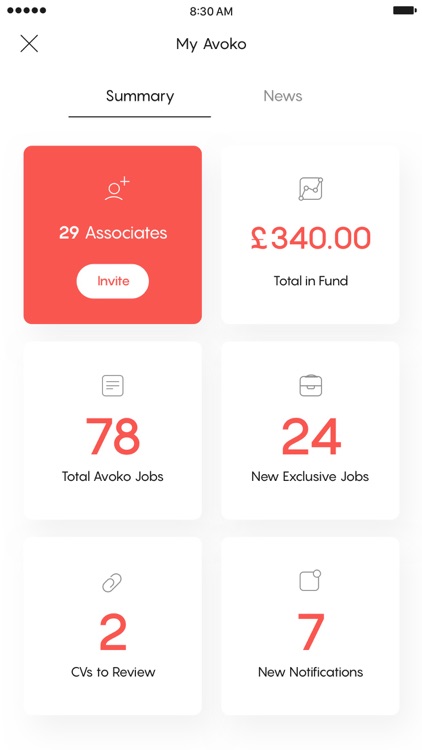The image is a screenshot taken from a phone. At the top left corner, there are five small black dots aligned horizontally. Centered at the top, the time reads "8:30 a.m." On the far right side, there is a solid black battery icon. Directly below the time, the text reads "my evoco."

Below "my evoco," there are two tabs: "Summary" on the left and "News" on the right. The "Summary" tab is underlined, indicating it is the active tab. Beneath the "Summary" tab, there is a red square containing the text "29 associates and invite," written in white. To the right of this red square, a white box displays "340 euros total in funds."

Further down, there are two more lines, each containing additional boxes. The first box displays: 
- "78 for jobs"
- "24 new exclusive jobs"
- "2 CVs to review"
- "7 new notifications"

The numbers in this section are written in red, while the box backgrounds are either white or red with white text.